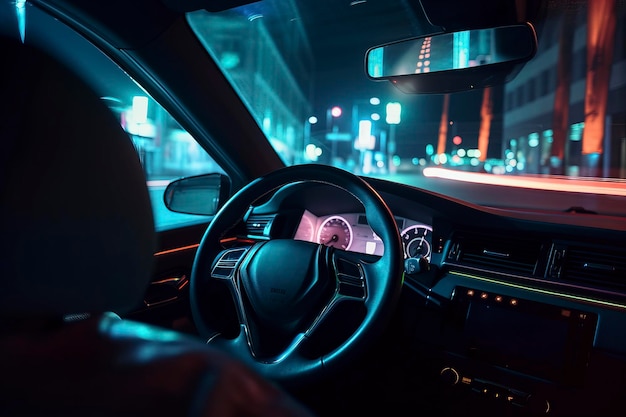The photograph captures a night-time scene from the interior of a car, likely taken from the passenger or back seat, facing the driver's seat, which is vacant. The overall interior is primarily black, with various dashboard lights providing illumination. The dashboard glows with purple lights, featuring distinct illuminated gauges, the speedometer or odometer, and the radio with glowing red dots above it. The steering wheel, also black, has three rows of buttons on the right side and two or three on the left. Below, the radio displays additional lit knobs, and there are vent registers for heating. Visible elements include the back and side of the headrest, the top of the driver's seat backrest, and the rearview mirror showing lights shining from behind. The front windshield reveals an indistinct cityscape with street lights and silhouetted buildings on both sides. The image is a rectangular, horizontally oriented photograph, emphasizing the nocturnal city center captured through the car's windshield.